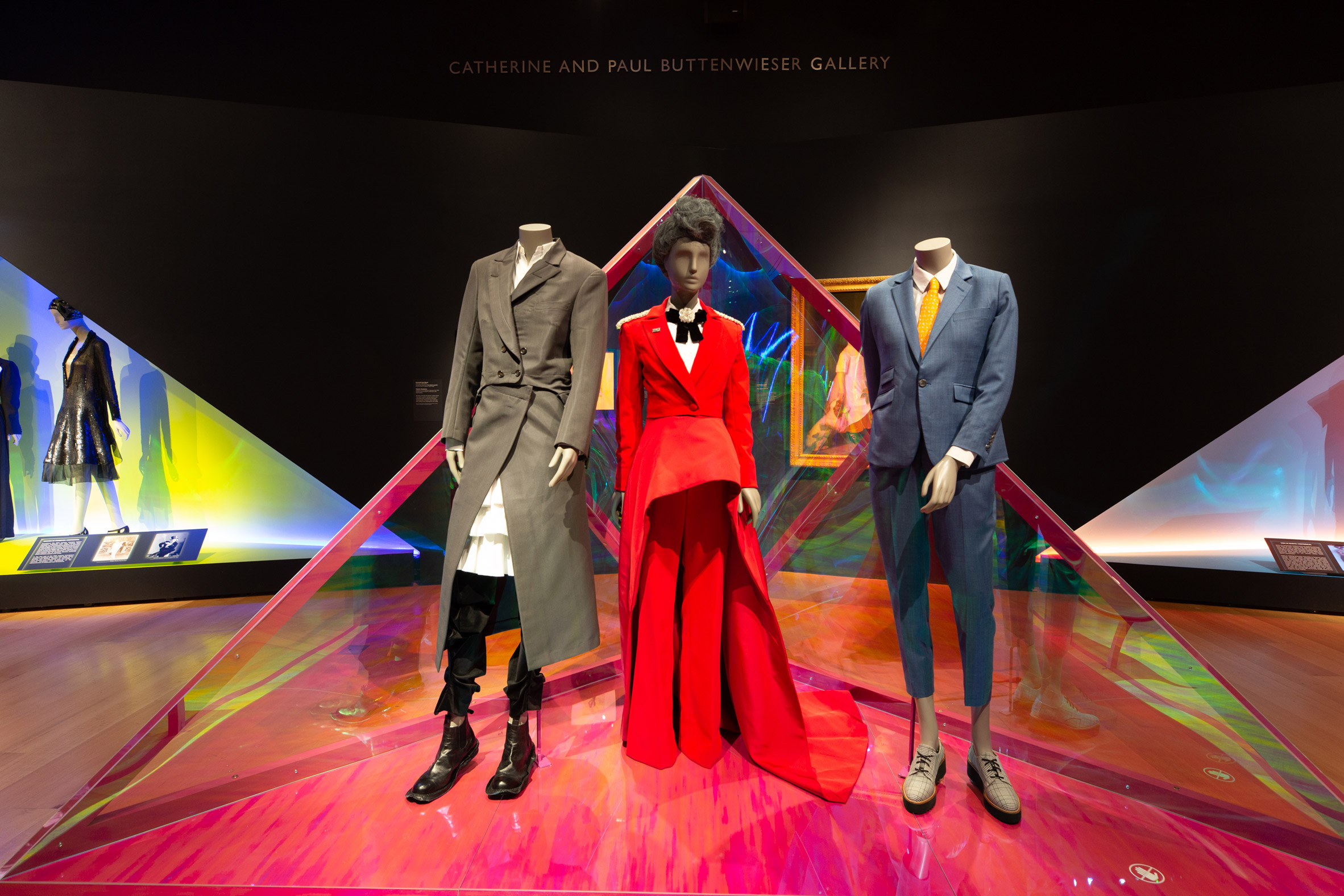This photograph, taken inside the Catherine and Paul Buttonwiser Gallery, captures a stunning fashion exhibit that treats clothing as art. The central focus is a trio of mannequins, prominently displayed within a pink, transparent, holographic plastic pyramid that's open on one side. The backdrop of the exhibit is a striking black inverted triangular wall, enhancing the dramatic presentation.

The middle mannequin, distinctly feminine with a coiffed hairstyle, is clad in a red tuxedo-like suit with a high-low skirt—short in the front and flowing long in the back—layered over red pants. This ensemble is paired with a white undershirt and a black bow tie. The left mannequin, headless, sports a taupe trench coat cinched at the waist, flared out, combined with a ruffled white skirt layered over satin black pants—creating an androgynous yet feminine look. Completing the trio, the right mannequin, also headless, is dressed in a slate blue suit with high-water trousers, a bright yellow tie, a white shirt, and beige shoes.

The gallery’s design features dramatic angles and additional triangular exhibits can be seen flanking the central display. This expertly curated exhibit underscores the intersection of fashion and art, inviting viewers to explore the intricate details and artistry of contemporary clothing design.